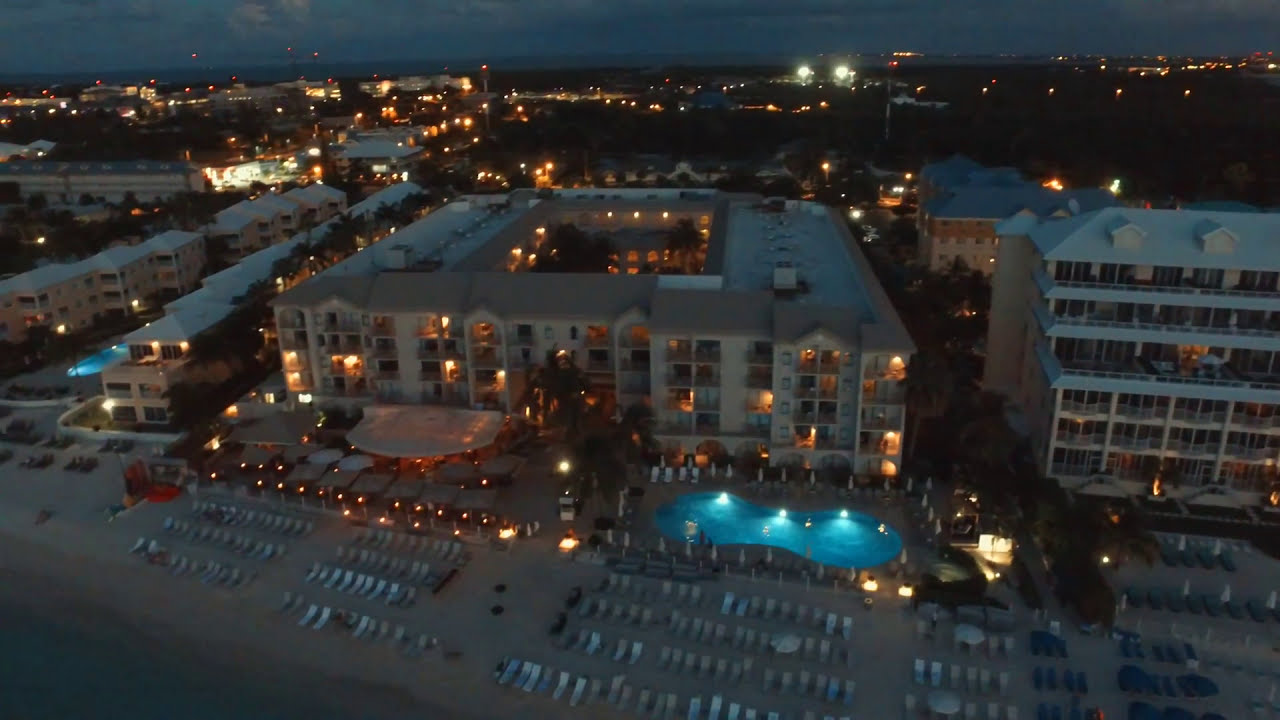Aerial nighttime photograph of a bustling beachfront resort. At the bottom of the image, a sandy beach is lined with rows of neatly arranged lounge chairs and bordered by the edge of dark blue water. Moving upwards, the central feature is a five-story resort building with a well-lit kidney-shaped swimming pool on its right side. This building is characterized by a central square courtyard and numerous balconies. Adjacent to it on the right is another multi-story condominium. Surrounding the central resort are several multi-story buildings with their lights illuminating the night, contributing to the vibrant atmosphere. Further into the distance, additional buildings with glowing windows dot the horizon, while the darkening sky above is tinged with deep blue hues and scattered clouds. The vivid colors in the image include tan, brown, white, light blue, red, orange, yellow, and black, adding to the overall realism and detailed representation in this drone-captured scene.